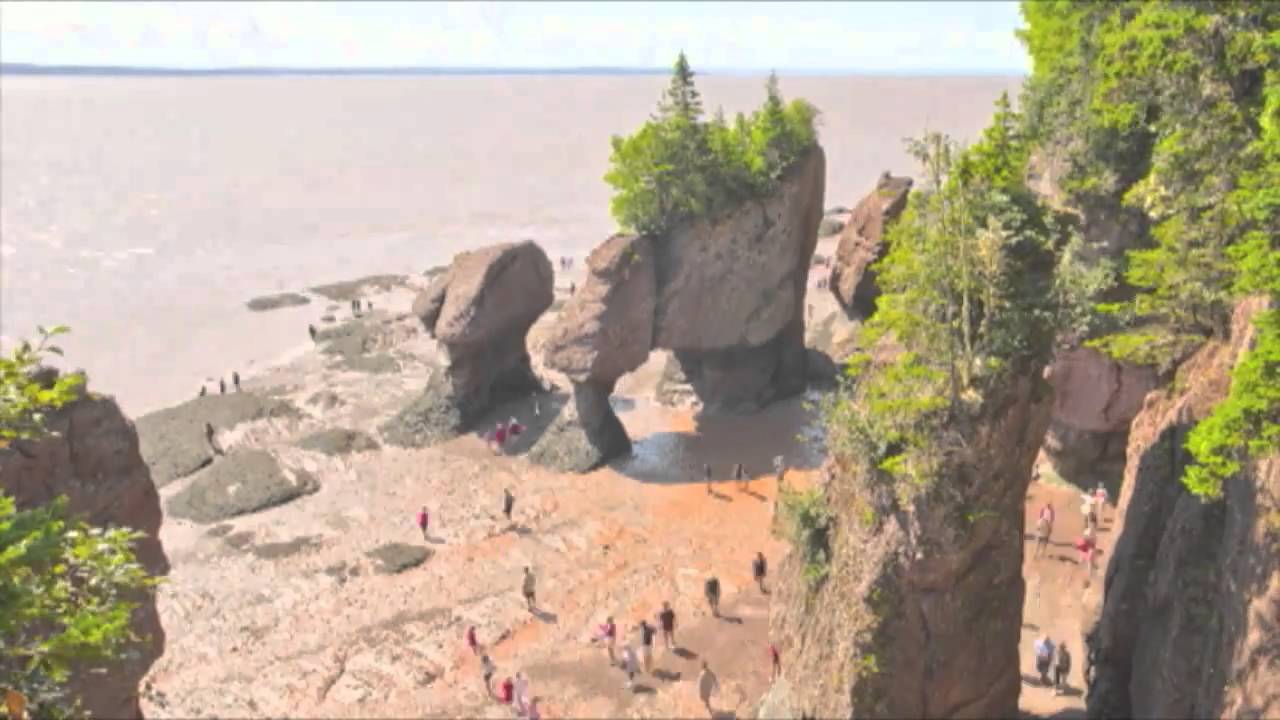This image appears to be a highly detailed and realistic artwork, perhaps a painting, depicting an aerial view of a rugged coastline that might lead to a beach or a large lake. Dominating the scene are striking rock formations that have eroded at their bases, creating mushroom-shaped columns, each unique and visually distinct from the others. On top of these formations, lush green vegetation and trees thrive, contrasting with the rocky surfaces below. 

The beach itself is covered in clay-colored mud, dotted with big boulders featuring patches of green growth. Tiny, indistinguishable humans populate the shore, wearing an array of red, white, and dark-colored shirts. They appear almost like obscured figurines, adding a sense of scale to the expansive landscape.

To the far left, a body of grayish water, likely an ocean, borders the beach, merging with the muddy shoreline. The sky above is a faint blue, adding a serene backdrop to the lively and complex terrain below. The right side of the image showcases mountains enveloped in greenery, while a cliff with vegetation stands prominently on the left. This visually compelling scene blends intricate natural elements with human activity, drawing the viewer into its enchanting and varied landscape.